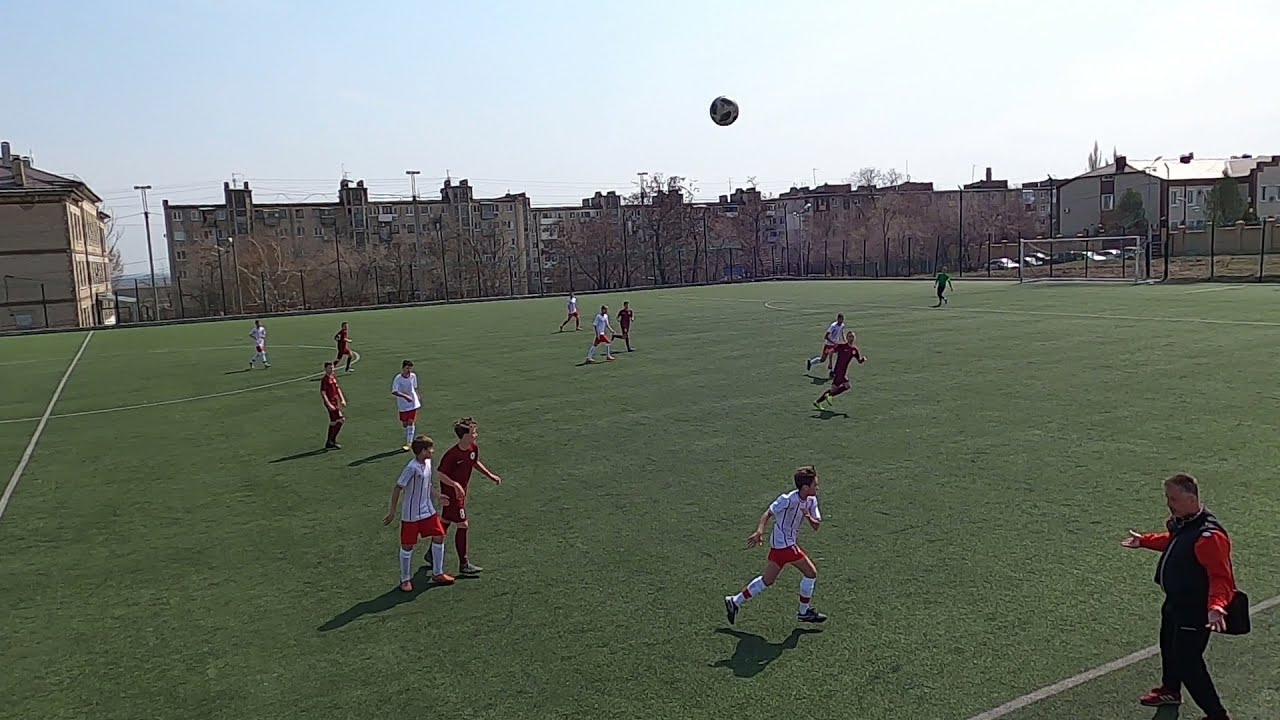In this vibrant daytime photograph, a dynamic youth soccer game unfolds on a lush green field encircled by a tall black fence. Two teams of young boys, seemingly of Caucasian descent, compete with one team donning white jerseys with black stripes, red shorts, and white socks, while the opposing team sports burgundy jerseys, shorts, and socks. A black and white soccer ball is captured mid-air near the center of the image, contrasting against the clear, light blue sky devoid of clouds.

On the lower right corner of the field stands a Caucasian coach, distinguishable by his short gray and brown hair. He wears a long-sleeve red shirt beneath a black vest, coupled with black pants and red shoes. His arms are extended to his sides with palms facing upward, appearing to express a frustrated or questioning gesture.

Beyond the soccer field, the background showcases rows of multi-story brick buildings that resemble apartments, adding an urban touch to the scene. The setting suggests a location that could be in Germany or London, emphasizing the European architectural influence.